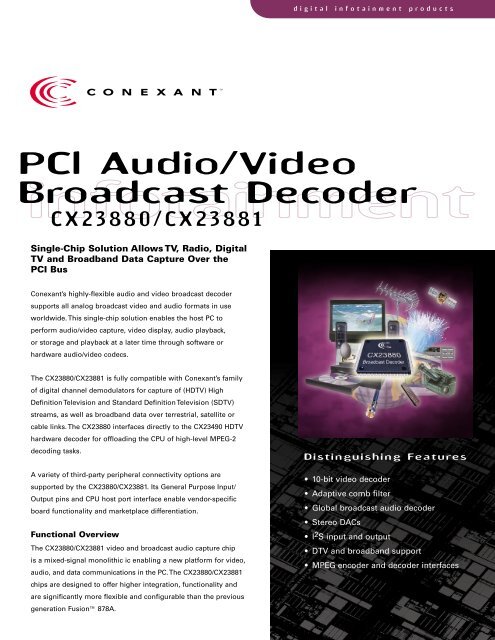This image is an advertisement with a clean white background, and it's designed to appear like an informational article. In the top left corner, there is a prominent logo consisting of three Cs nested within each other, followed by the company's name, "Conexant," in black text. Adjacent to this logo is a small purple banner stating "Digital Infotainment Products." 

The headline reads "PCI Audio Video Broadcast Decoder" in bold black letters, followed by the model numbers "CX23880/CX23881." Underneath, smaller bold text explains, "Single chip solution allows TV, radio, digital TV, and broadband data capture over the PCI bus."

The main text consists of three detailed paragraphs along the left-hand side of the ad, alongside a smaller bold section titled "Functional Overview," accompanied by another descriptive paragraph. To the right, there is a black rectangle containing an image of a computer chip set against a background imagery of various computer hardware items, such as a monitor, satellite, and camcorder.

Above this image, in white text, is a list titled "Distinguishing Features," outlining the product’s key capabilities. The listed features include:
- 10-bit video decoder
- Adaptive comb filter
- Global broadcast audio decoder
- Stereo DACs
- PS input and output
- DTV and broadcast support
- MPEG encoder and decoder interfaces